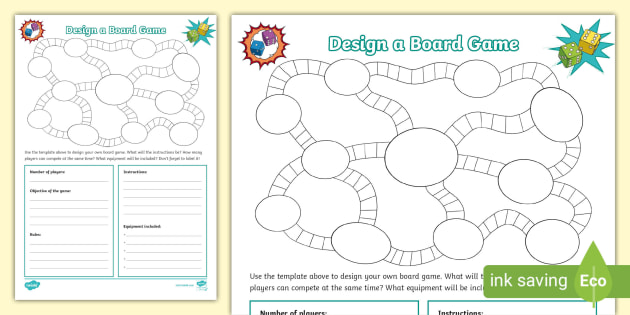The image features a comprehensive template for designing a board game, prominently labeled "Design a Board Game" at the top. The main section is dotted with elliptical circles connected by lines, forming a detailed game diagram. In the upper left corner, a blue and red die is set against an orange and red circular background, while the upper right corner shows a blue and yellow die on a blue star background. The bottom half of the template includes blank lines within green-bordered boxes for filling out game details such as the number of players, instructions, and equipment needed. The bottom right of the template features a green rectangle with the text "Ink Saving Eco" inside a green leaf icon. On the right side of the composite image, there's a zoomed-in view of the board game outline, and beneath it, partially visible text instructs users to "Use the template to design your own board game. What will ... Players can compete at the same time? What equipment will be ..." The rest of the text is obscured by the eco-friendly logo.